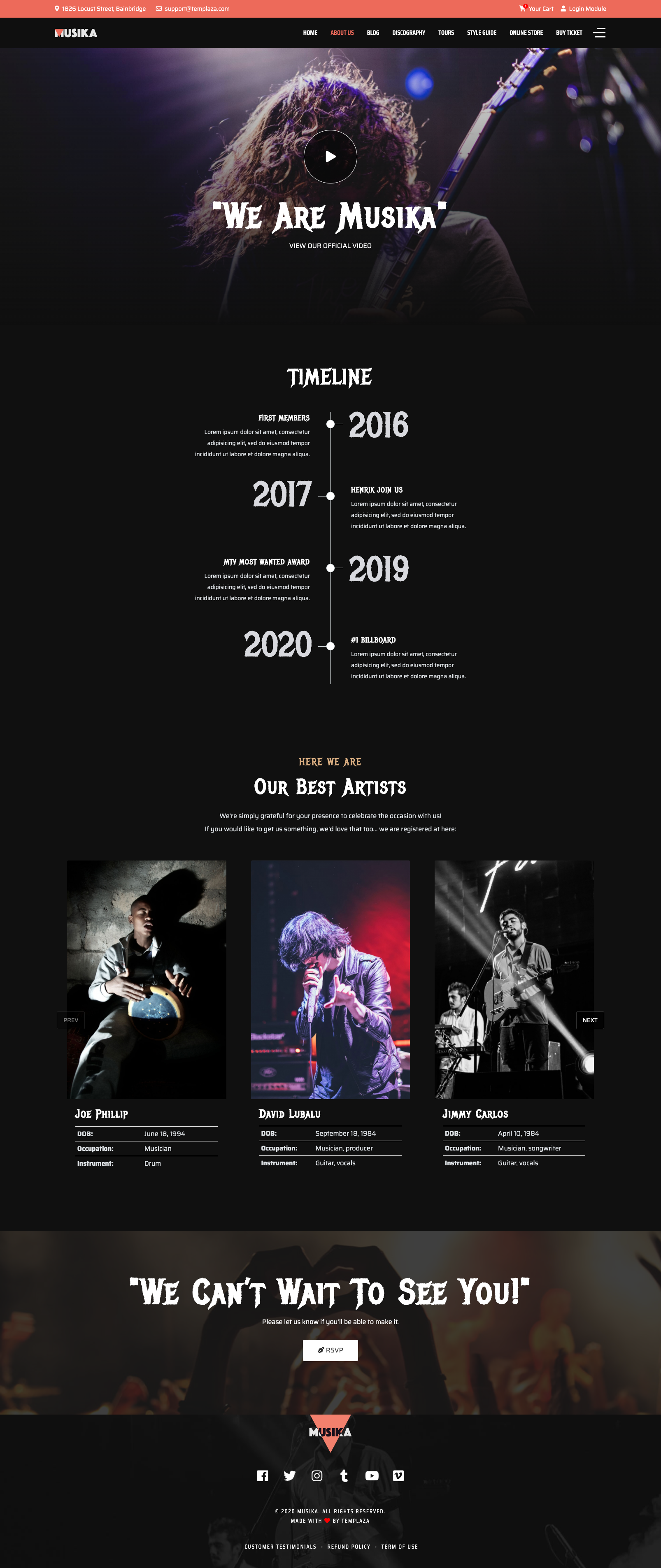This image appears to be a screenshot from the website Tempasa.com, featuring various details about the band Lusika. At the top, there's a male icon, and the banner displays the address "1826 Locust Street, Bainbridge." To the right, you can see the "cart" and "login" modules. A black banner with the word "Lusika" stretches across the page, and below it are menu items including "Home," "About Us," "Blog," "Discography," "Tours," "Style Guide," "Online Store," and "Buy Ticket," all written in white.

Below this menu, there is a prominent section announcing "We are Lusika" with an invitation to view their official video. This section features an image of a man with long hair holding a guitar, with a play icon superimposed over his head.

Further down, a timeline tracks the band's history: 
- "First Members" in 2016, 
- "Henrik joins us" in 2017,
- "MTV Most Wanted Award" in 2019, and
- "#1 Billboard" in 2020.

The bottom section introduces the band's members:

1. **Joe Philip**
   - **Date of Birth:** April 10, 1984
   - **Occupation:** Musician, Songwriter
   - **Instruments:** Guitar, Vocals

   Joe, pictured on the right, is playing a guitar.

2. **David Lupo**
   - **Date of Birth:** September 18, 1984
   - **Occupation:** Musician, Producer
   - **Instruments:** Guitar, Vocals

   David, in the middle, is shown singing with long dark hair and wearing a leather jacket.

3. **Jimmy Carlos**
   - **Date of Birth:** June 18, 1984
   - **Occupation:** Musician
   - **Instrument:** Drum

   Jimmy, on the left, is depicted as an African dark-skinned male playing a drum-like instrument.

The bottom section of the image contains a message inviting fans to celebrate the band's presence and details about registering for gifts. The text concludes with "We can't wait to see you. Please let us know if you'll be able to make it. RSVP."

Finally, the footer displays "Lusika" with an orange triangle in the center, alongside icons for Facebook, Twitter, Instagram, and other platforms, followed by "2020 Lusika. All rights reserved. Made with love by Tempasa." Below that are links to "Customer Testimonials," "Refund Policy," and "Terms of Use."